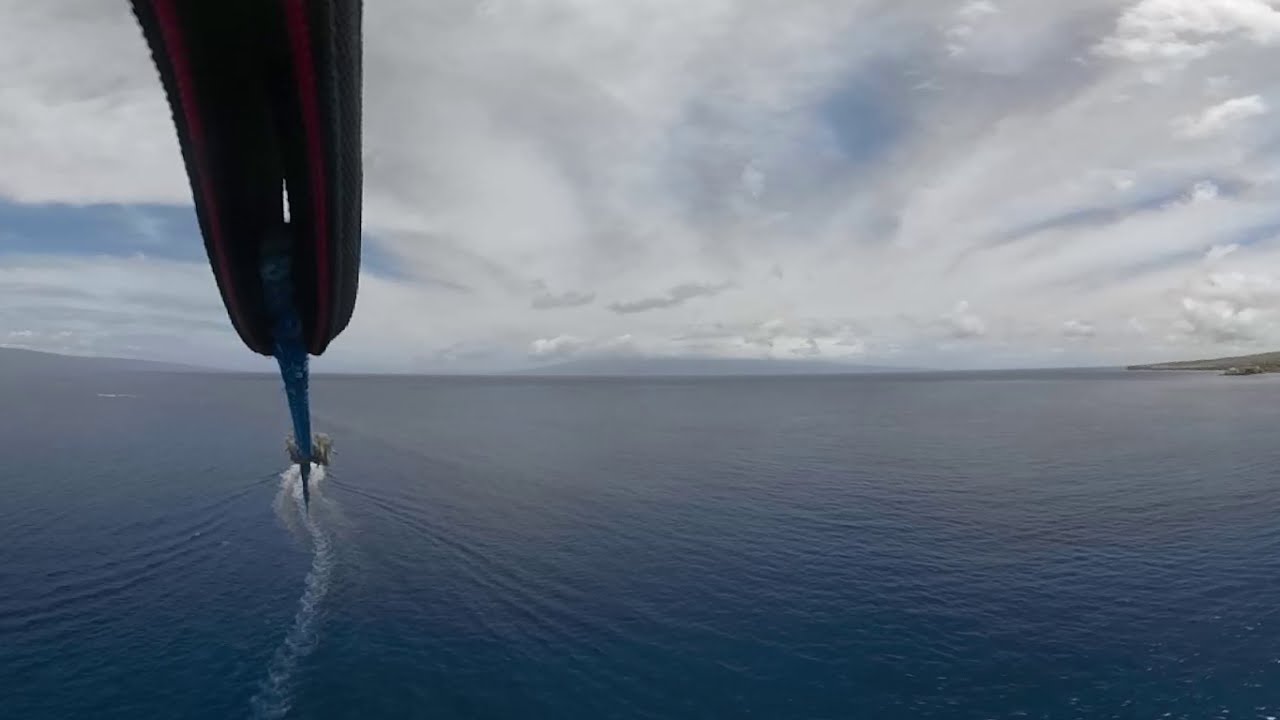The daytime outdoor image showcases a vast body of dark blue water spanning to the horizon, with some land faintly visible on the very far right edge. A partially obscured boat travels through the water, leaving waves in its wake and hinting at pulling a rope or an indistinct dark object behind it. At the top left corner of the image, a curved metal device with a pointy end dangles and appears to touch the water, creating ripples. The sky is predominantly cloudy, with patches of partial blue, casting a gray-blue tone over the scene.